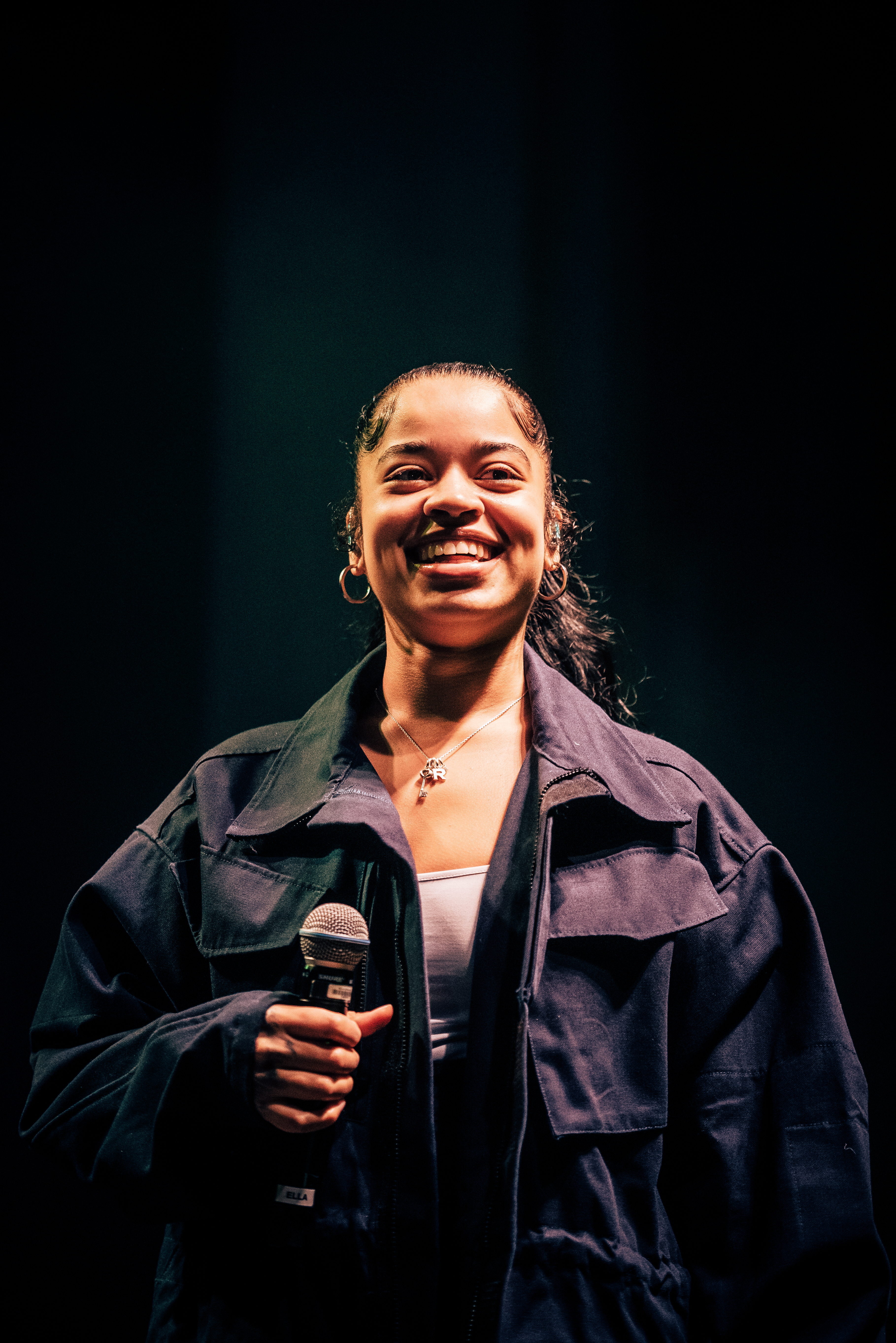The photograph features a young black woman, likely in her college years or early adulthood, beaming with a wide, genuine smile while holding a microphone in her left hand. She is dressed in a stylish black leather jacket with a thin grey tank top underneath. Her dark, wavy hair frames her face, and she accessorizes with gold hoop earrings and a necklace. The woman exudes confidence, appearing upbeat and happy under clear lighting that suggests she might be performing or speaking. The background is a solid black, drawing all attention to her radiant presence in the image.